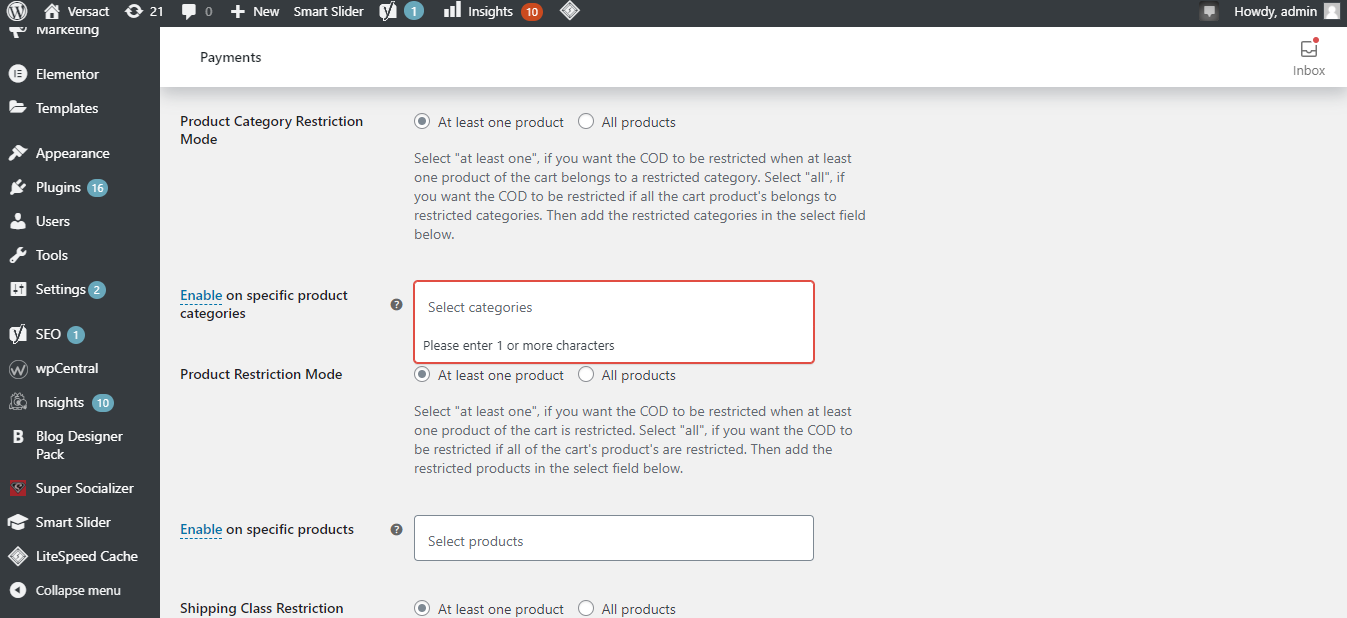The screenshot depicts the dashboard of a website, labeled "Veristat." The interface features several administrative options and metrics, primarily on a dark background with white text. 

On the left side, a vertical menu displays various sections: Marketing, Elementor, Templates, Appearance (with a notification indicating 16 items), Users, Tools, Settings (with 2 items), SEO (with 1 item), WP Central, Insights (with a red circle showing 10 items), Blogger Design Pack, Super Socializer, Smart Slider, Lightspeed, Cache, and a Collapsible Menu.

In the top-right corner, the screen reads "Howdy, Admin," indicating the user is logged in. Below the top bar, the main content area appears to be focused on Payments. This section is underlined by a white band featuring the word "Payments" in black text. 

Two highlighted modes are displayed: Product Category Restriction Mode, indicated by a red box around "Select Categories" with instructions to enter one or more characters and click the "At Least One Product" button, and Product Restriction Mode, which is enabled for specific products.

Additionally, there are icons and statistics including a green circle with a '1', a red circle with '10', and the number '21' next to a refresh icon, located towards the left-hand side of the interface.